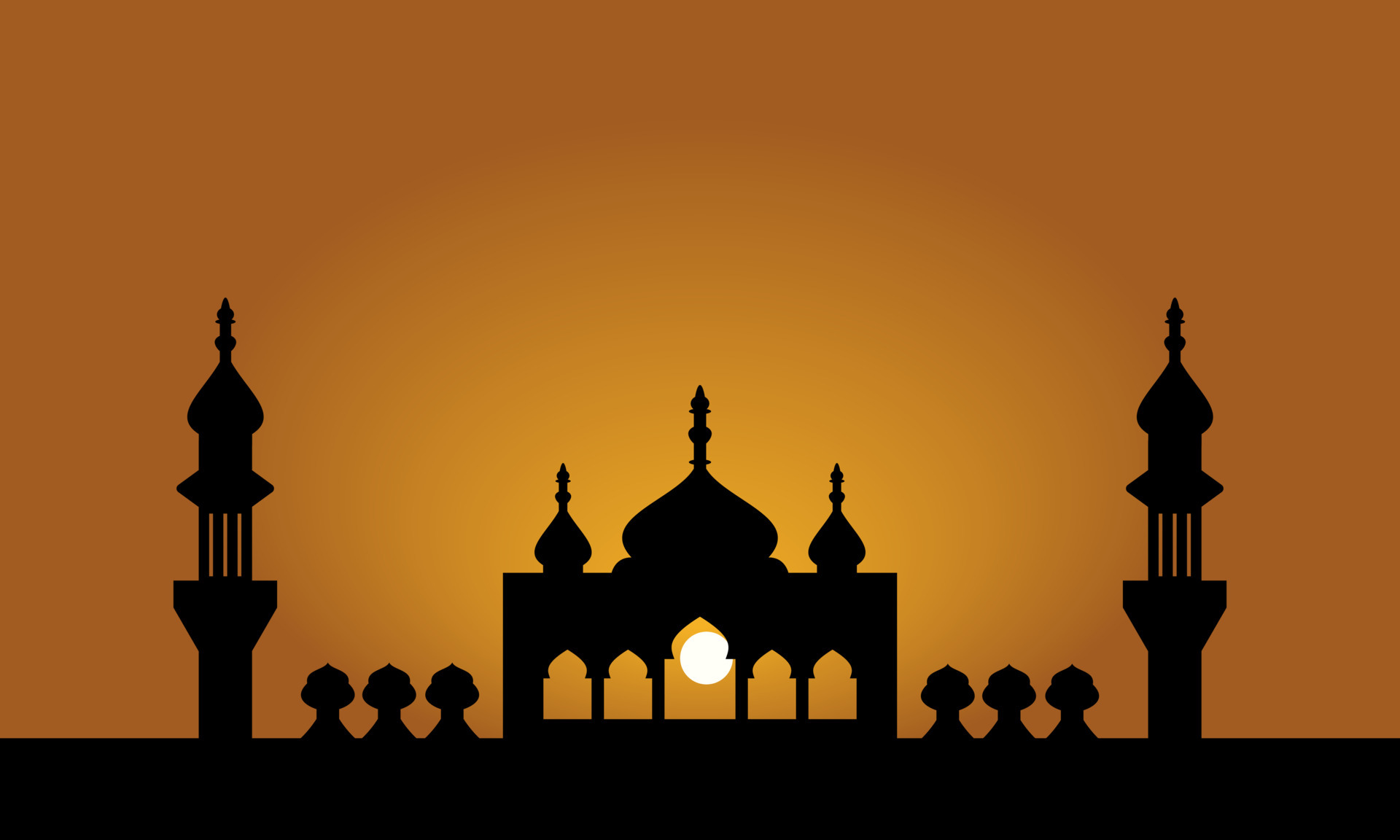This image is a detailed, computer-generated vector illustration depicting a serene sunset scene with an architectural silhouette reminiscent of mosques in South Asia or Indonesia, similar to the Taj Mahal. The background features a gradient from a vivid orange at the edges to a lighter yellow near the center, simulating the warm hues of a setting sun just above the horizon. Dominating the foreground is a black silhouette of a grand structure. 

At its center stands a large rectangular building with five cutout arches, the middle one larger than the rest, allowing the warm glow of the sun to pierce through and illuminate the architectural details. Atop this central building are three steeple-like spires, the tallest in the middle, flanked by smaller ones resembling elongated Hershey's Kisses with pointed tops. Flanking this central structure are pairs of minaret-like towers on both sides, each adorned with slender spires, evocative of delicate toothpicks on the heads of the towers. The entire architectural ensemble sits on a solid black bar, representing the ground, which anchors the magnificence of the scene against the vast expanse of the colorful sky.

The symmetry of the composition, with mirroring buildings and detailed silhouettes, captures the intricate beauty and harmony typical of classical Islamic architecture. The image as a whole presents a tranquil and mesmerizing visual of a twilight horizon, blending the simplicity of silhouette art with the rich visual appeal of a sunset sky.